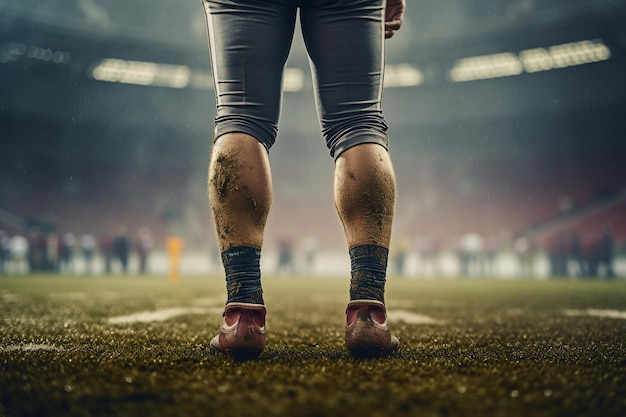The image captures the lower half of an athlete, likely a football player, during a sporting event. The focal point is the athlete's mud-splattered calves, exposed from the back of his knees to his ankles. He is dressed in tight, gray capri-like pants with a stripe down the side, which are pulled up just below the knees. Covering his legs are tall, dark gray socks, also streaked with mud, and bright red cleats firmly planted on a flat, astroturf surface. The background is blurred but reveals the outlines of numerous spectators, suggesting a bustling stadium atmosphere. The venue features rounded stands with red seating, and overhead lights pierce through a somewhat smoky or foggy environment, enhancing the dramatic ambiance of the scene.